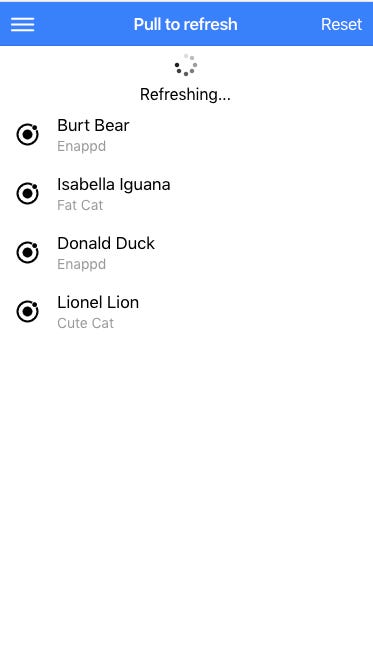A cropped screenshot of what appears to be a game character list displayed on a white background. At the top of the screen is a blue bar featuring the text "Pull to Refresh" in large white letters at its center. The word "Reset" appears in white on the far right of the bar, while a white menu icon is situated on the far left.

Beneath the blue bar, centrally located, is a loading icon composed of partially colored dots arranged in a circle. Directly below this loading icon, the word "Refreshing" in bold black letters is displayed, followed by an ellipsis.

Continuing downward, there's a vertical list of players, each accompanied by an icon to their left. The icons consist of a small black circle with a large black-and-white outlined circle surrounding it. Four users are listed:

1. Bert Bear, labeled as "inapt" in small gray letters.
2. Isabella Iguana, labeled as "Fat Cat" in small gray letters.
3. Donald Duck, labeled as "inapt" in small gray letters.
4. Lionel Lion, labeled as "Cute Cat" in small gray letters.